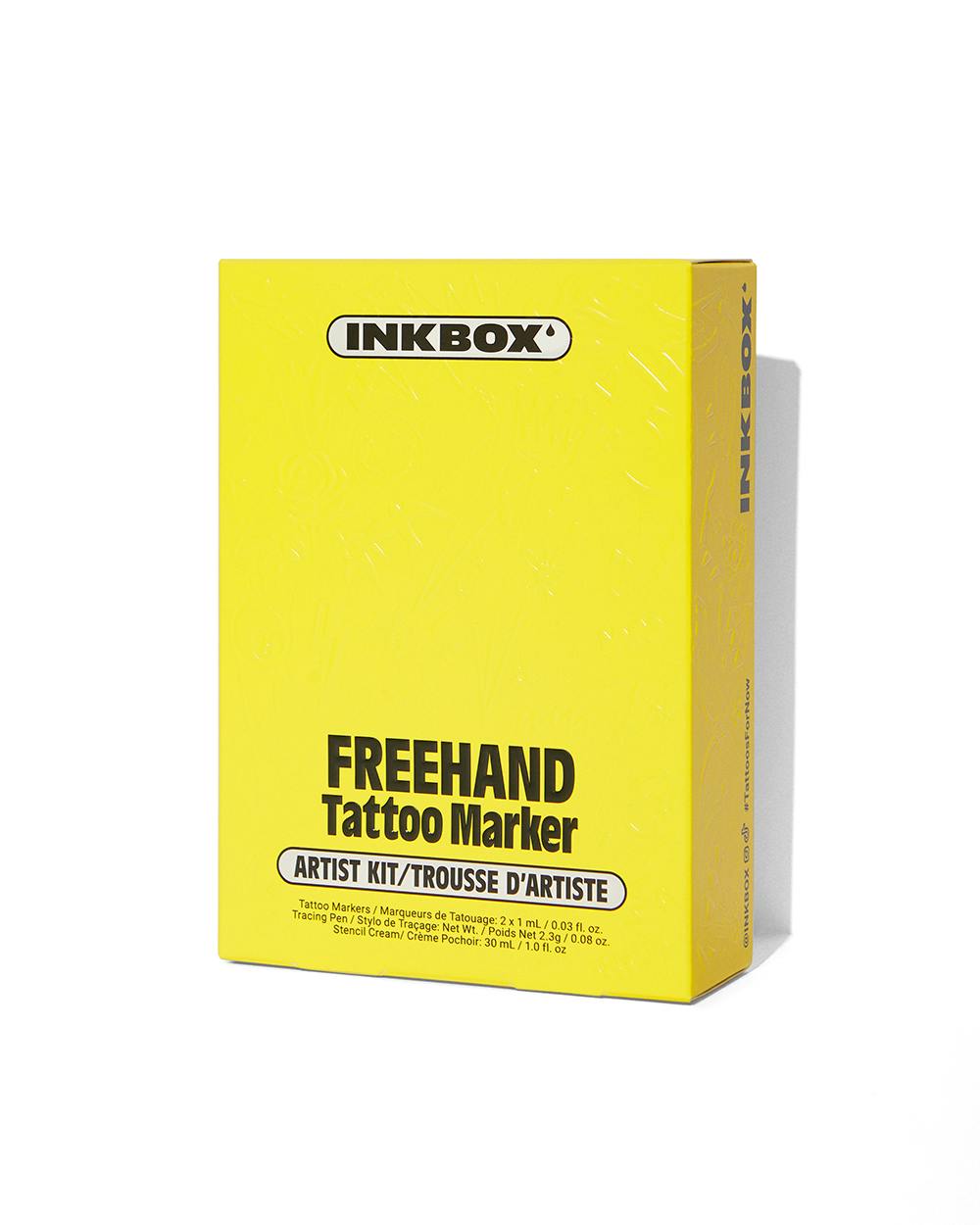The photograph features a yellow, rectangular cardboard box sealed in plastic, standing upright against an entirely white background. The box casts a subtle shadow to the right. At the top of the box, a white oval section displays the words "Ink Box" in bold black lettering, complemented by a small black water droplet design as part of the logo. Below, the text "Freehand Tattoo Marker" is prominently written in bold black letters. Further down, another elongated white oval section reads "Artist Kit / Trace the Artist" (interpreted as possibly being bilingual, with "Traus De Artist" in French). The fine print at the bottom lists the contents as "Tattoo Markers, Tracing Pen, Stencil, Cream," alongside measurements provided in milliliters and ounces. On the side of the box, the brand name "Ink Box" is repeated, coupled with several lines of smaller text likely containing copyright information.